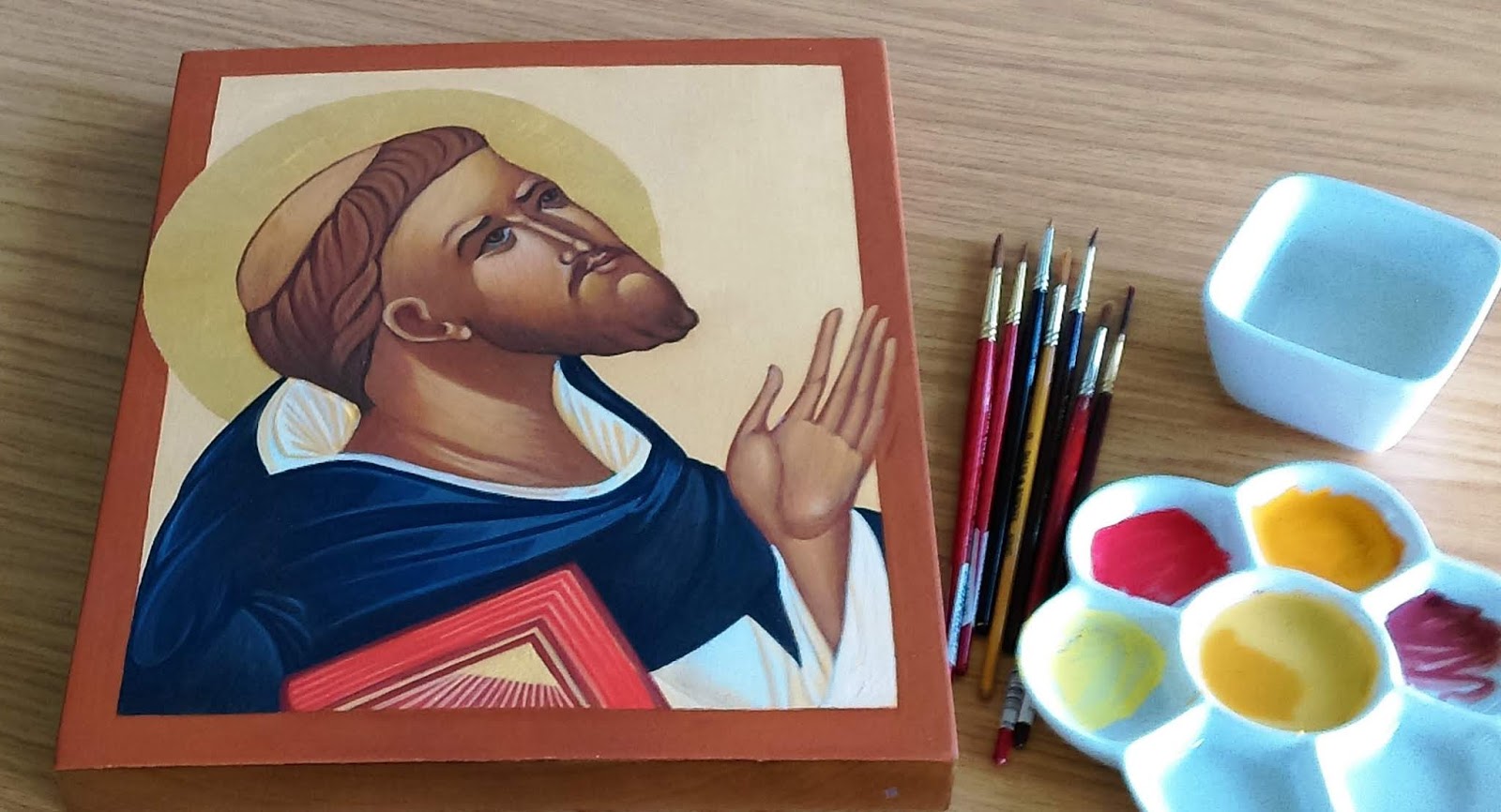The image depicts an artist's workspace featuring a detailed watercolor painting of a saint, set against a light beige wooden desk. The saint, portrayed from the chest up, has a balding head with brown, curly hair circling his scalp, and a beard. He dons a white robe with a blue sash draped over his shoulders, holds a red book with his right hand, and raises his left palm upwards. A pale yellow halo accentuates his head, and he gazes upward and to the right. This rectangular painting rests on a brown block or canvas.

Adjacent to the painting on the right, there is an array of seven thin paintbrushes, each identified by different colors including red, blue, and yellow. Further right lies a white ceramic palette resembling a flower, with seven compartments—six outer ones circling a central one—filled with various shades of watercolor paints, including yellow, dark yellow, light yellow, pink, purple, and two different blues. Above this colorful palette, a square white ceramic bowl is filled with clear water, serving as an essential tool for the painting process.